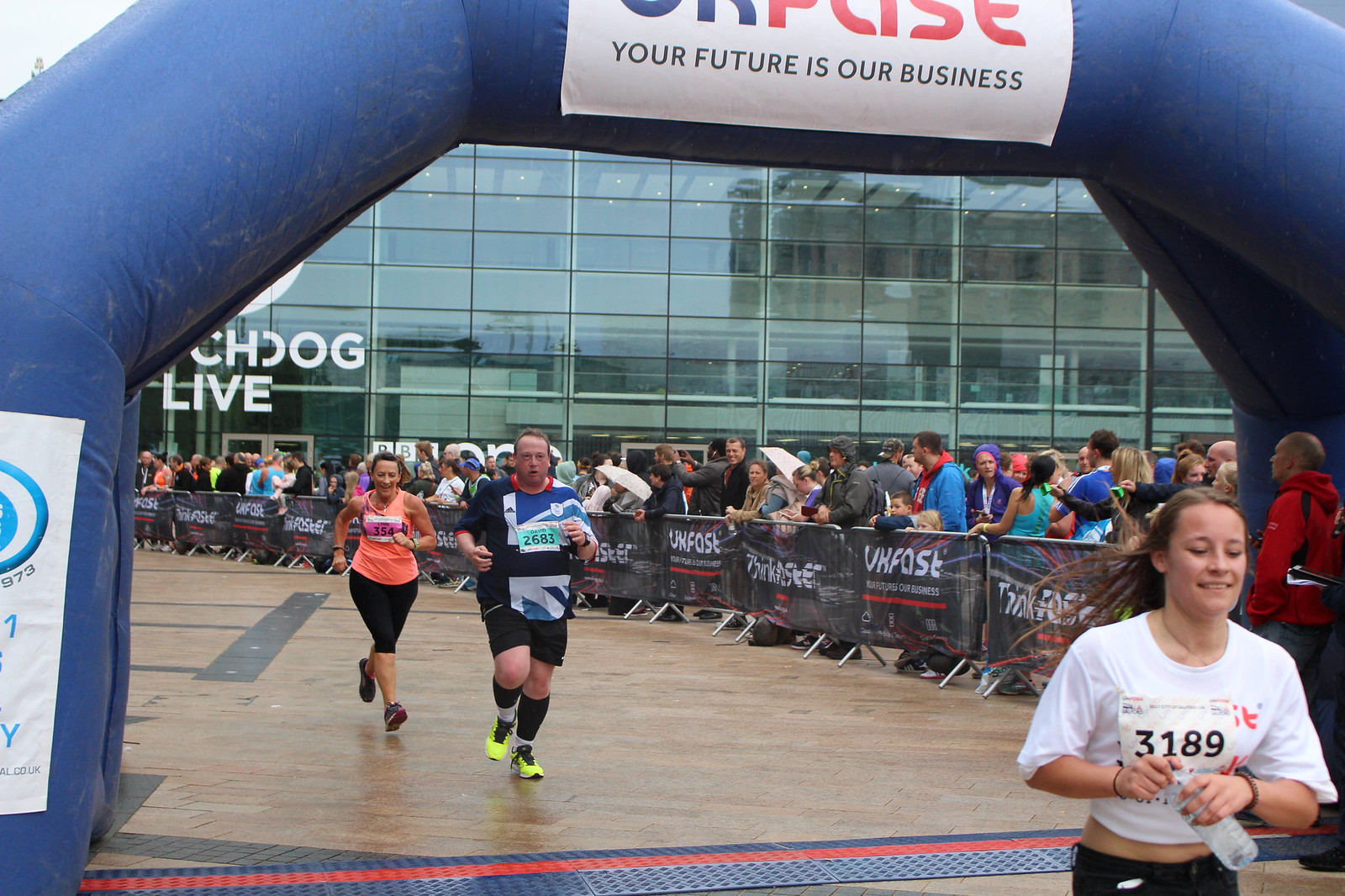The image captures a bustling corporate marathon event, prominently featuring a striking glass-walled corporate office building in the background with partially visible signage that includes phrases such as “CH dog life” and “your future is our business.” A distinctive brown wooden plank pathway with black patterns stretches towards the foreground, bordered by barricades adorned with banners reading “VK fast” and “your future is our business.” 

In the midst of the race, three runners are prominently visible. In the forefront, a young woman with the number 3189 is sporting a white short-sleeved top and holding a plastic water bottle. Close behind her is a clean-shaven man wearing a black and blue T-shirt with the number 2683, paired with black shorts, socks, and neon green sports shoes. Trailing him is another runner, a woman dressed in an orange sleeveless top numbered 354, complemented by black leggings and black sports shoes.

The racecourse culminates in a blue inflatable overhead structure serving as the finish line, emblazoned with the slogan “your future is our business.” Spectators, shielded against the rain with umbrellas and ponchos, line the barricades beside the path, their excitement adding to the vibrancy of the occasion. The presence of additional logos like "BBC" and a large crowd comprising men, women, and children further accentuate the lively and well-attended nature of this event. Near the finish line stands a person in a red hoodie, possibly assisting with the race logistics.